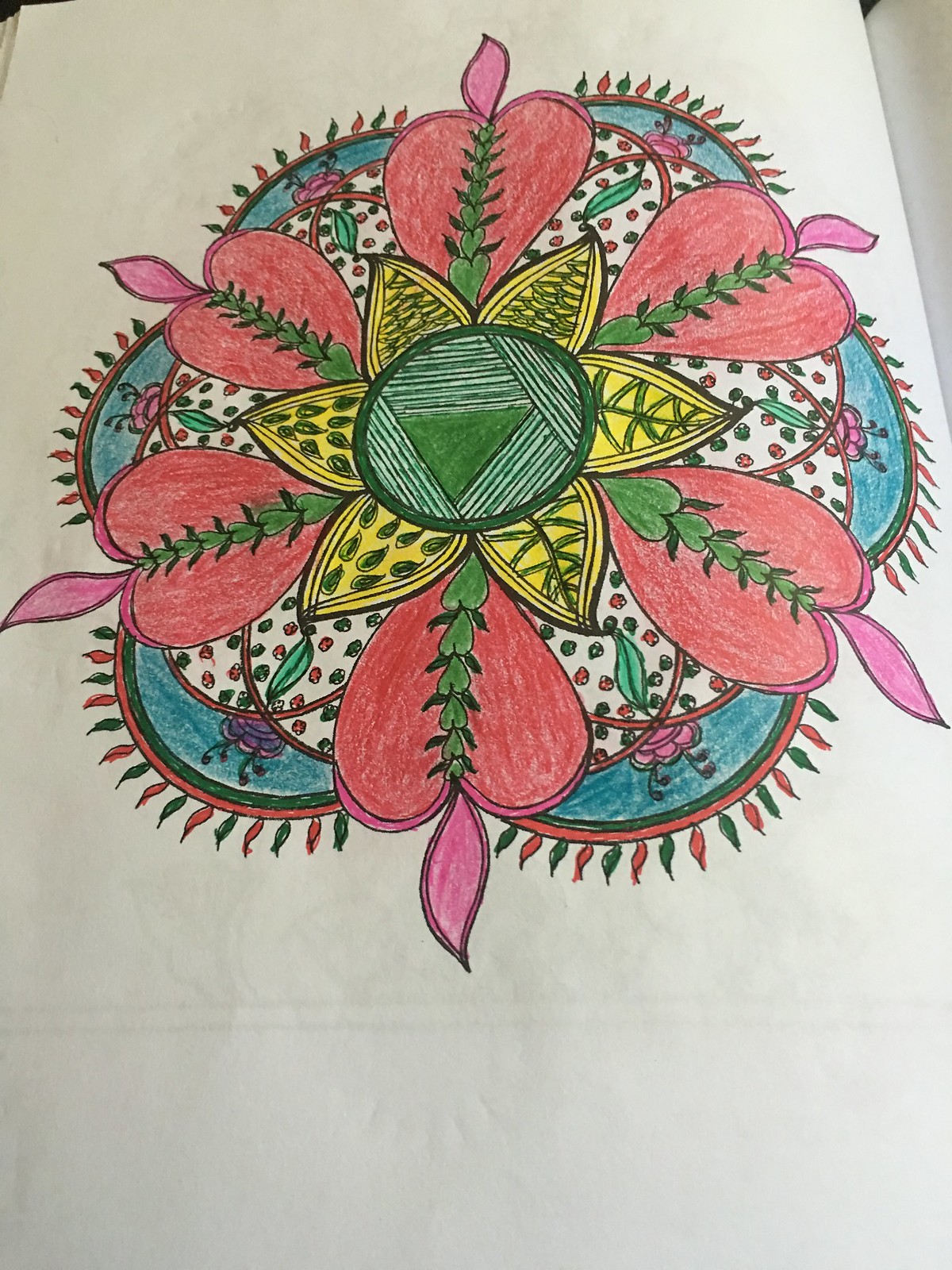The image is a color photograph of a sophisticated and detailed colored pencil drawing on a white piece of paper, possibly part of a notebook or fabric like a tablecloth. The vibrant, large, circular floral design occupies almost the entire surface of the medium and is centered perfectly. The design's focal point is a central green triangle encircled by green stripes. Radiating from this center are six yellow petals decorated with intricate green designs. Beyond these are six elongated, heart-shaped red petals, each featuring a central green tendril and topped with a delicate pink flourish reminiscent of an apple core. At the outer layer, there are additional curved blue petals detailed with red and green edges, along with small red and green leaves. The entire composition is set against a blue and white area adorned with tiny floral patterns, and more delicate, pink petals are arranged around the periphery, forming an intricate and visually striking mandala-like pattern. The faint grey visible under the drawing suggests another design on the reverse side of the page. Small background details, such as tiny black areas, hint at the notebook's presence beyond the drawing.